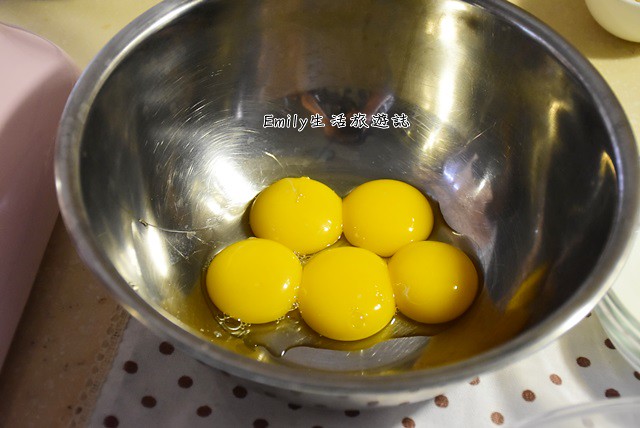This detailed photograph, taken indoors, captures a close-up view of five separated egg yolks nestled in a shiny, stainless steel mixing bowl. The yolks are arranged with three on the bottom row and two slightly above them. The bowl, which prominently features the name "Emily" followed by Asian characters (likely Chinese or Kanji) in black lettering with a white border, reflects the inverted image of the photographer. Resting on a light brown countertop with speckles of brown and white, the bowl sits atop a white cloth adorned with small brown polka dots. Surrounding the setup, there are partially visible objects, including a pink purse to the left and some indeterminate items towards the right, contributing to the food preparation environment.